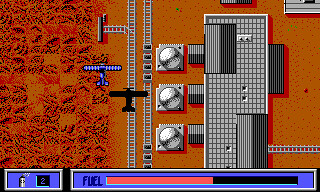The image appears to be a screenshot from a video game, captured from an aerial perspective. The primary focus is on two airborne planes set against a burnt orange backdrop. The first plane is blue, and cast beneath it is a black shadow mimicking its shape, creating a striking contrast against the orange ground. The blue plane seems to be navigating along visible white tracks presumably on the terrain below.

On the right side of the screen, three silver knobs are arranged vertically, each connected to a different section of a long, flat-roofed silver building. This structure features a covered walkway linking various parts of the building. Additionally, a silver sphere is perched atop one of the roofs, adding further detail to the scene.

The bottom of the screen displays a blue rectangle bordered in white, labeled "Fuel." A pink bar within this box indicates that the fuel level is currently at approximately 50%. This intricate composition of visual elements suggests a dynamic and engaging gameplay environment.